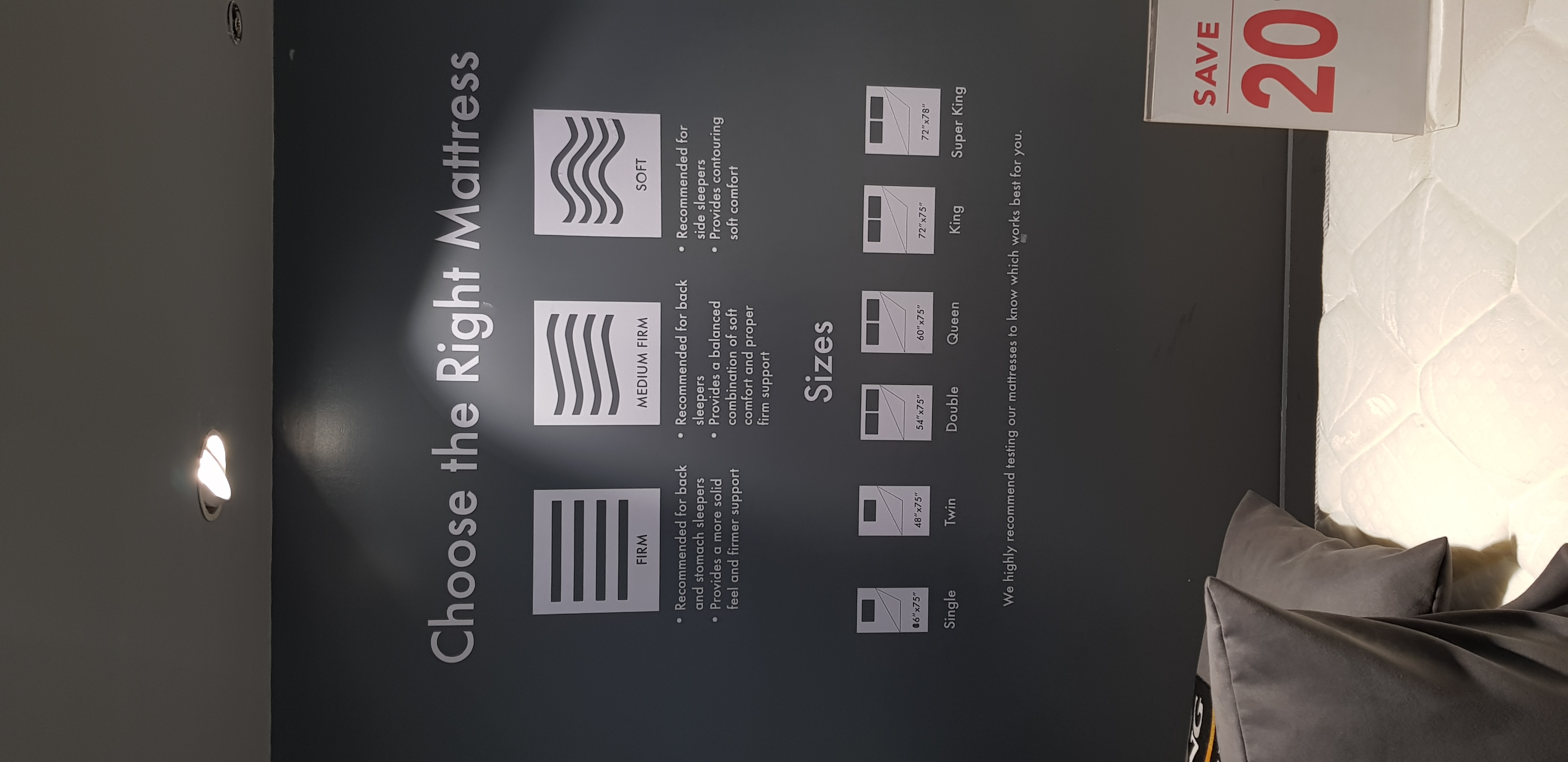This color photograph, captured inside a furniture store, prominently features a meticulously organized display wall. The wall, painted a sophisticated dark gray, is adorned with crisp white lettering bearing the directive "Choose the Right Mattress." Below this heading, three distinct squares illustrate the varying mattress firmness options: Firm, Medium Firm, and Soft. Further down, the display provides detailed information on mattress sizes, showcasing six smaller panels labeled Single, Twin, Double, Queen, King, and Super King. Emphasizing the event, the bottom right corner of the wall boasts a "Save 20%" promotional message, signaling an ongoing sale. In the foreground, a neatly-made mattress with plush pillows invites shoppers to experience comfort firsthand.